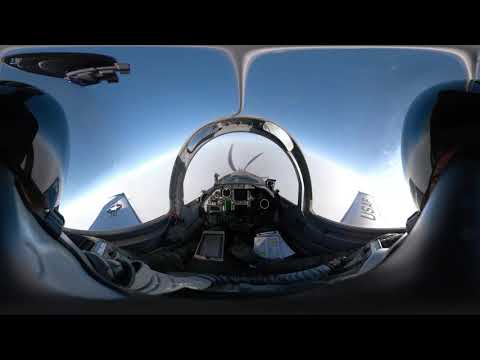The image depicts the interior of a gray US jet cockpit during flight, as seen from a pilot's point of view. The two-seater cockpit features two individuals, both wearing black helmets with visors and gray uniforms, seated in gray chairs. The left and right sides of the image show the pilots' helmets and control panels that exhibit black and green buttons. A black and silver apparatus is positioned above the left pilot's seat. In front of them, the windshield reveals a clear blue sky with white clouds, and the nose of the plane is visible with two silver propellers spinning. The front wings, visible through the windshield, bear distinct markings: the right wing shows the letters "US" while the left wing features a star logo. The cockpit itself contains various complex control panels and devices, including a laptop-like tablet and multiple instruments, surrounded by silver, white, and gray surfaces.